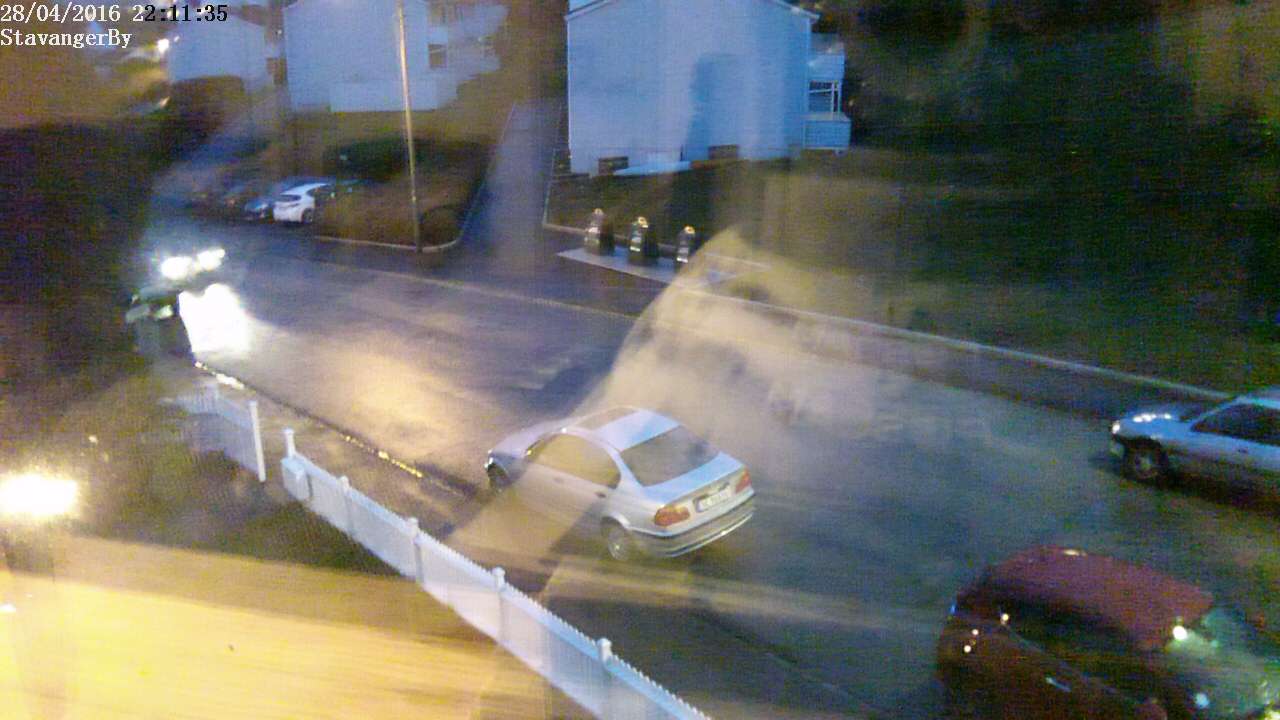The image appears to be a low-resolution, blurry photograph taken with a digital camera through a window, likely at night. Visible in the bottom-left corner of the image is a flash, contributing to various reflections that obscure the view slightly. In the top-left corner, there is a timestamp showing "28 April 2016, 23:22:35." Outside the window, a street scene is partially visible with a few cars on the road, one of which has its headlights on. There are houses in the upper center-left portion of the image, and a considerable amount of greenery is visible in the top right. A fence runs diagonally from the center-left to the bottom left of the frame. Reflections suggest an indoor setting, possibly a living room, adding to the complexity of the image.